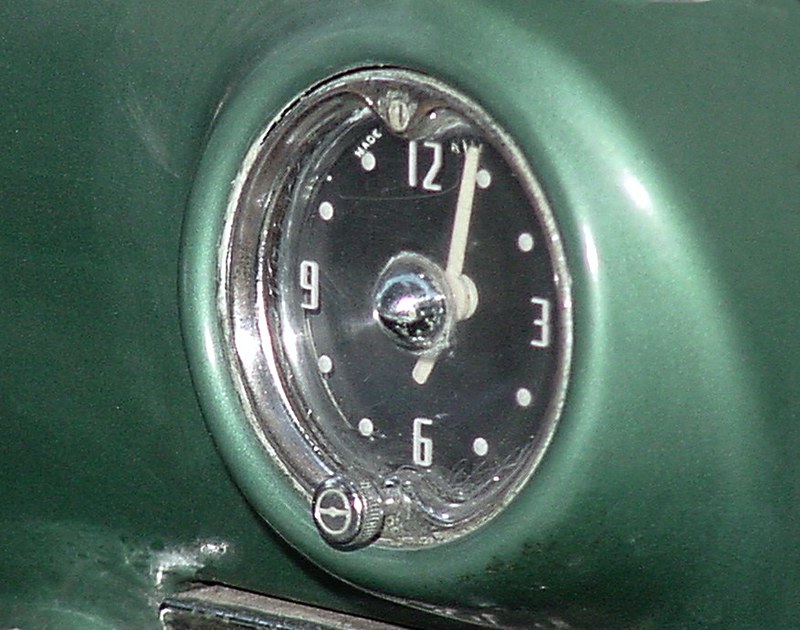This detailed image captures a close-up of a dashboard dial, likely from a car. The surrounding area is adorned with a sophisticated green metallic paint that exudes a luxurious appeal. The dial itself is constructed from metal and is embedded into a slightly elevated section of the dashboard, adding a dimensional quality to the setup. The dial's face is a deep black, providing a stark contrast to the crisp white numerals that denote the positions of 12, 3, 6, and 9 o'clock. Fine English text is inscribed on the upper portion of the dial, and while it's challenging to read all the details, the word "MADE" is discernible, indicating information about the dial's origin or manufacture. At the bottom of the dial, there is a knob designed for adjustments, adding to the dial's functionality and precision.